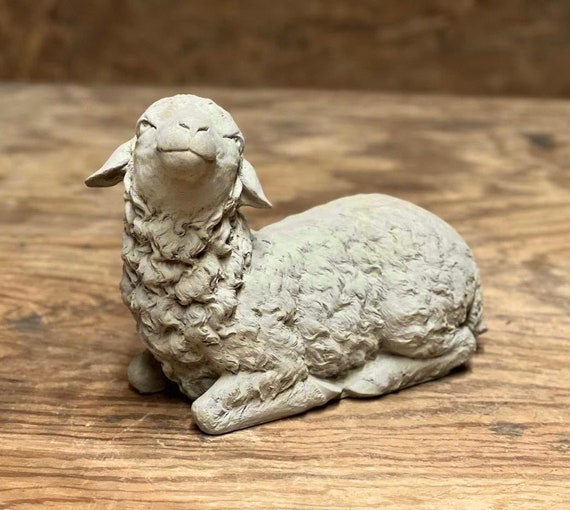The image showcases a detailed ceramic figurine of a young lamb, positioned on an old, worn wooden surface with visible scratches and age-related stains. The lamb is depicted lying down with its legs curled beneath it, giving an impression of tender relaxation. Its face is angled upward and slightly to the left, presenting a subtle, gentle smile, with narrow eyes and long, floppy ears that hang down. The texture of the lamb's wool is intricately crafted, capturing the realistic curls and waves that imitate the softness and appearance of real wool. In the blurred background, there is a hint of a carpet or possibly grass, adding to the composition's depth. The overall ambiance suggests the photo was taken during the daytime, with the sculpture placed prominently at the center and foreground of the image.